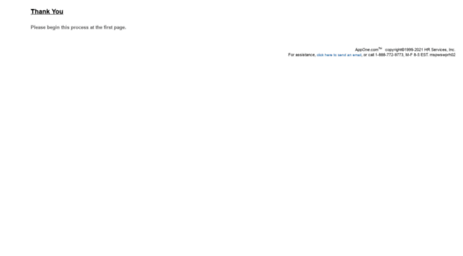Here is a possible cleaned up caption for the image described:

"The image captures a nearly blank webpage from AppleCare.com. In the upper left-hand corner, the word 'Thank you' is prominently displayed in bold, underlined black text. Below it, there is a prompt to log in to the previous page. The webpage's background is stark white, making the minimal text hard to discern. At the bottom right, partly obscured numbers are visible near a blue link offering email assistance. The page appears to be a final landing page, possibly confirming a purchase of an Apple product, and stands out for its lack of content, creativity, and even the presence of an Apple logo."